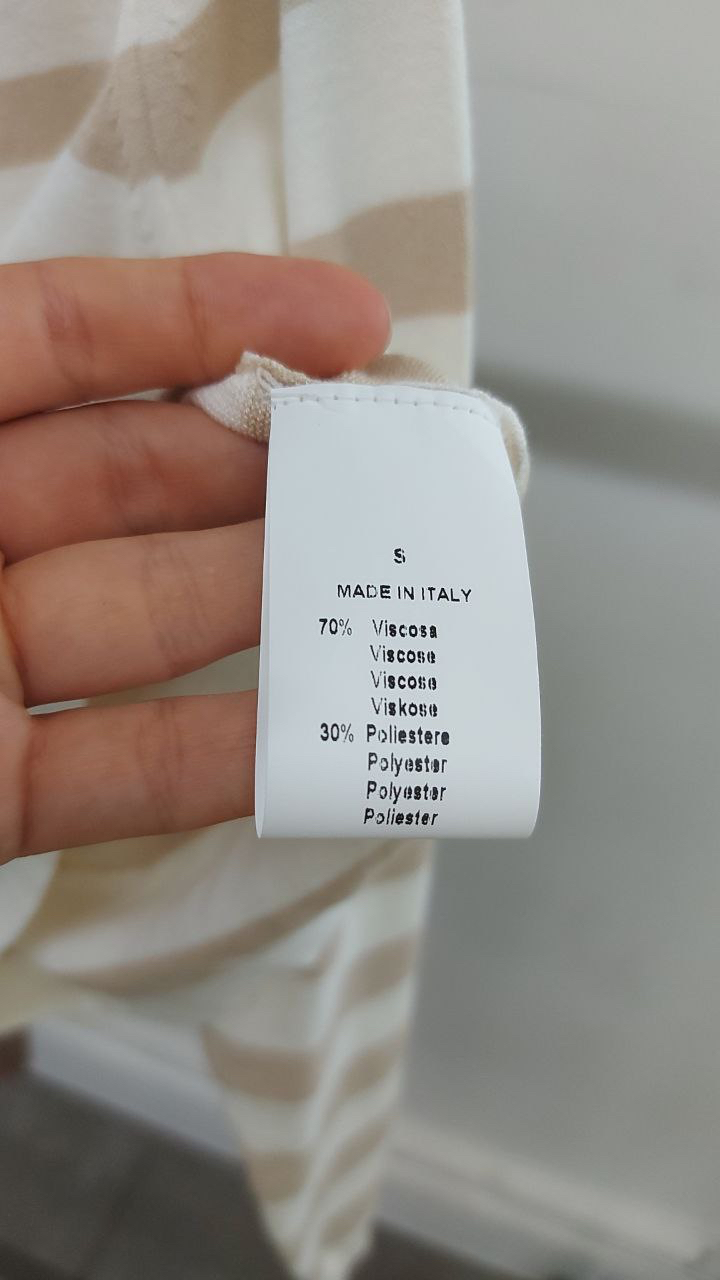This detailed color photograph portrays a close-up of a clothing label being held between the fingers of a person with medium white skin. The label, which is white with black print, is prominently displayed between four fingers positioned towards the center and left edge of the image. The label details include the letter "S," an indication that the garment is "Made in Italy," and the materials listed as "70% viscose" and "30% polyester," each presented in various languages. The background of the image reveals a blurred glimpse of the clothing item itself, which features grey and beige stripes. Additionally, the setting includes a greyish wall on the right side, decorated with grey skirting boards at the bottom. A dark grey horizontal line, possibly a shadow, aligns with the top of the clothing label. The floor beneath the scene is also dark grey, adding to the tonal coherence of the backdrop.